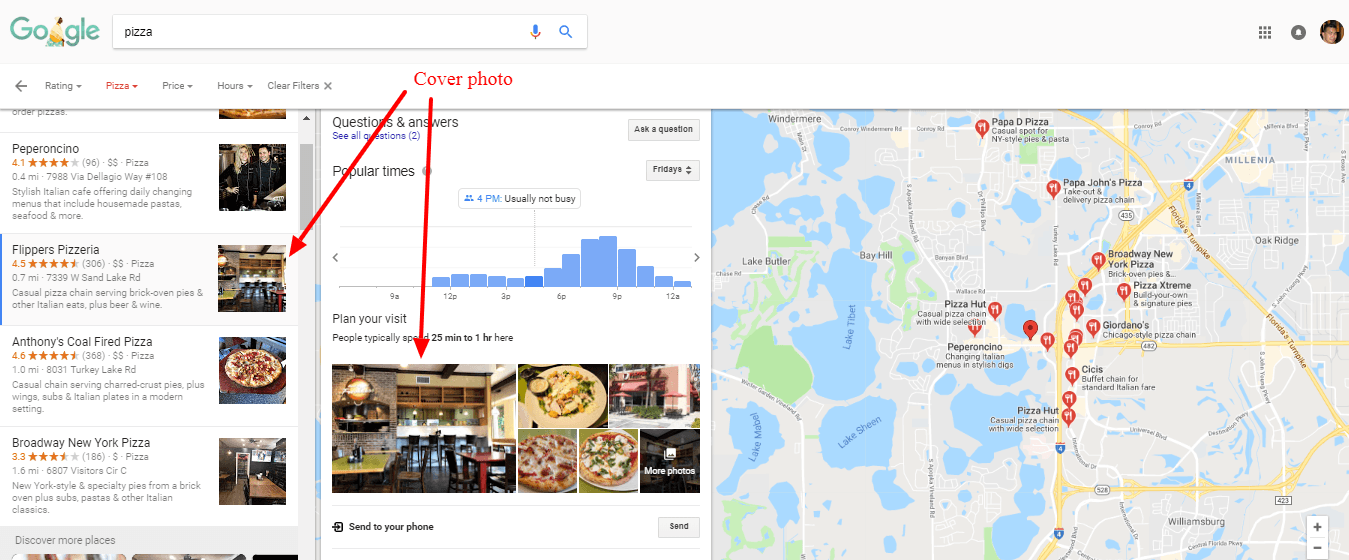A Google search results screenshot for the keyword "pizza" is displayed. The left side of the page lists various pizza places, each with accompanying ratings and descriptions. The top search result is "Pepperoncino," rated at 4.1 stars, featuring a picture of a chef in a black outfit. Below it, "Flipper's Pizzeria" is shown with a 4.5-star rating and a description of its casual dining atmosphere. 

Further down, "Anthony's Coal-Fired Pizza" is highlighted with an impressive 4.8-star rating and an enticing image of a pizza. Conversely, "Broadway New York Pizza" holds a lower rating of 3.3 stars. Adjacent to these listings, a map on the right indicates the locations of these pizza establishments.

The search results also offer filters for ratings, opening hours, and other criteria, plus an option to clear these filters. Additional information provided includes questions and answers about popular visitation times, helping users plan their visits efficiently.